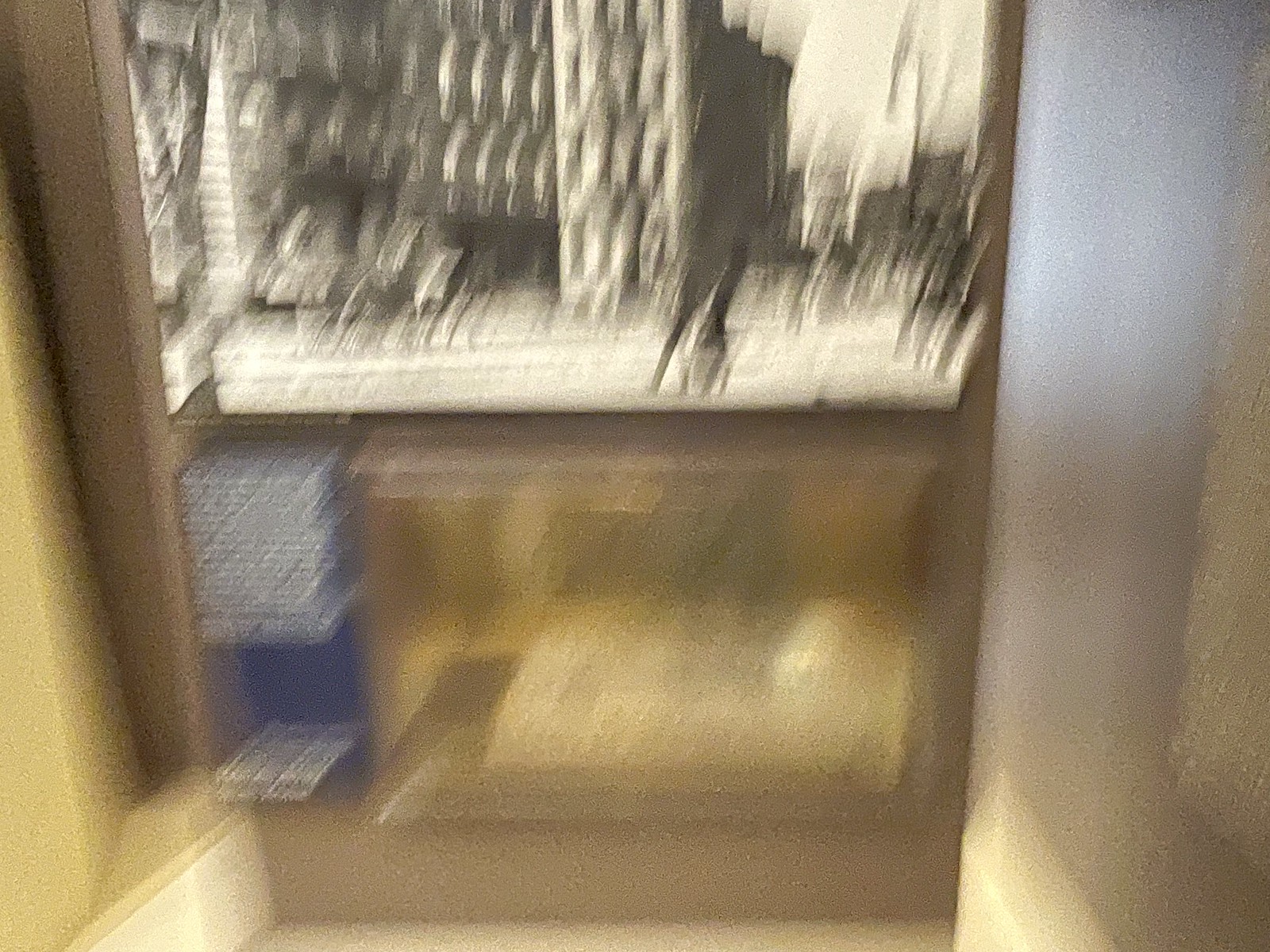Captured within the dim interior of what seems to be a museum, this photograph exudes an air of historical intrigue, despite its grainy and unfocused nature. Dominating the composition is a large, framed black-and-white image, seemingly depicting a grandiose building surrounded by several pedestrians in the foreground, which hints at an urban scene from a bygone era.

Beneath this central photograph, a blue-colored section catches the eye, likely a panel or placard intended to contextualize the display. To the right of this blue segment, another indiscernible shape appears, adorned with hints of yellow, though its exact nature remains elusive due to the image's lack of clarity.

Overall, the photograph provides a tantalizing glimpse into a possible historical exhibit, where the centerpiece black-and-white image invites viewers to explore the tales of architecture and human activity from another time, complemented by descriptive text likely presented in the blue section below.